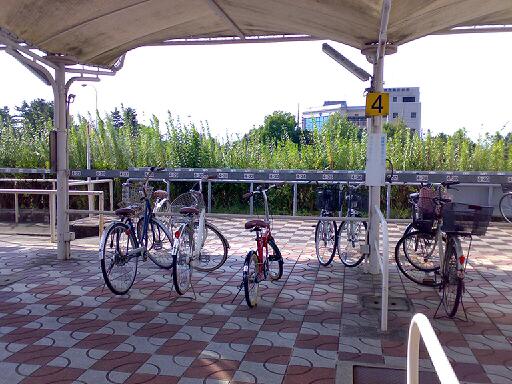In this outdoor daytime scene, we see a rectangular photograph featuring a group of bicycles parked under a canopy. The covered area, adorned with a light and dark gray checkered tiled floor, provides shade for the parked bikes. The ground is paved and lined with lush green trees, tall grass, and various plants in the distance, creating a verdant backdrop. A series of neatly arranged bicycles occupies this space, with around five visible facing in one direction and two facing the other. The bicycles showcase a variety of colors, including a notable red-framed bike with tall handlebars, a white one, and a blue and silver one. One of the dark-colored bicycles on the right is equipped with a basket in the rear. Near the back of the image, a silver metal bike rack and some empty racks can be seen, and a railing, possibly leading to a staircase, is also visible. In the far distance, a sizable building rises against a light blue, cloudy sky.